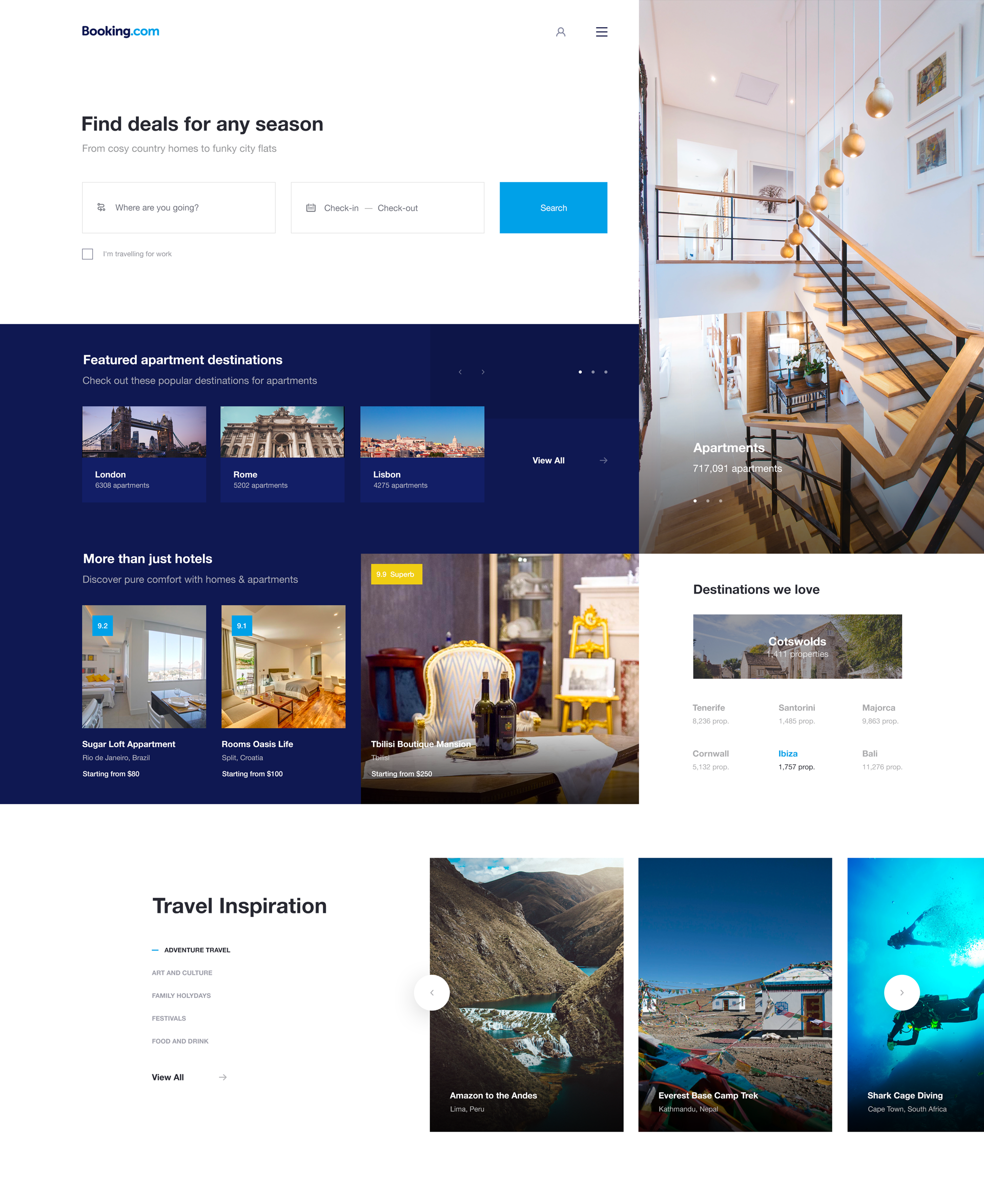This image captures a full-page view of the Booking.com website, offering a comprehensive snapshot without the need for scrolling. The top left corner features a prominent white box with "Booking.com" displayed in bold letters at the top. Just below, bold black text reads, "Find deals for any season," followed by a text box inviting users to enter a destination. Adjacent to this are fields for selecting travel dates and a large blue "Search" button.

Beneath this search section lies a significant blue banner adorned with thumbnails showcasing various travel destinations. On the right side of the screen, there's a large vertical rectangular image depicting the interior of a rental property available on Booking.com, complete with informative white text positioned at the bottom left of the photo. Below this vertical image is a small white box labeled "Destinations we love," listing multiple appealing locations.

At the bottom of the page, a section labeled "Travel Inspiration" appears on the left, presenting a vertical list of travel destinations with an option to "View all" at the bottom. To the right, three large rectangular thumbnail images feature different travel locales, accompanied by a white bubble that allows users to scroll through additional photos.

Overall, this webpage layout is designed to inspire travel while providing an intuitive user interface for planning trips.